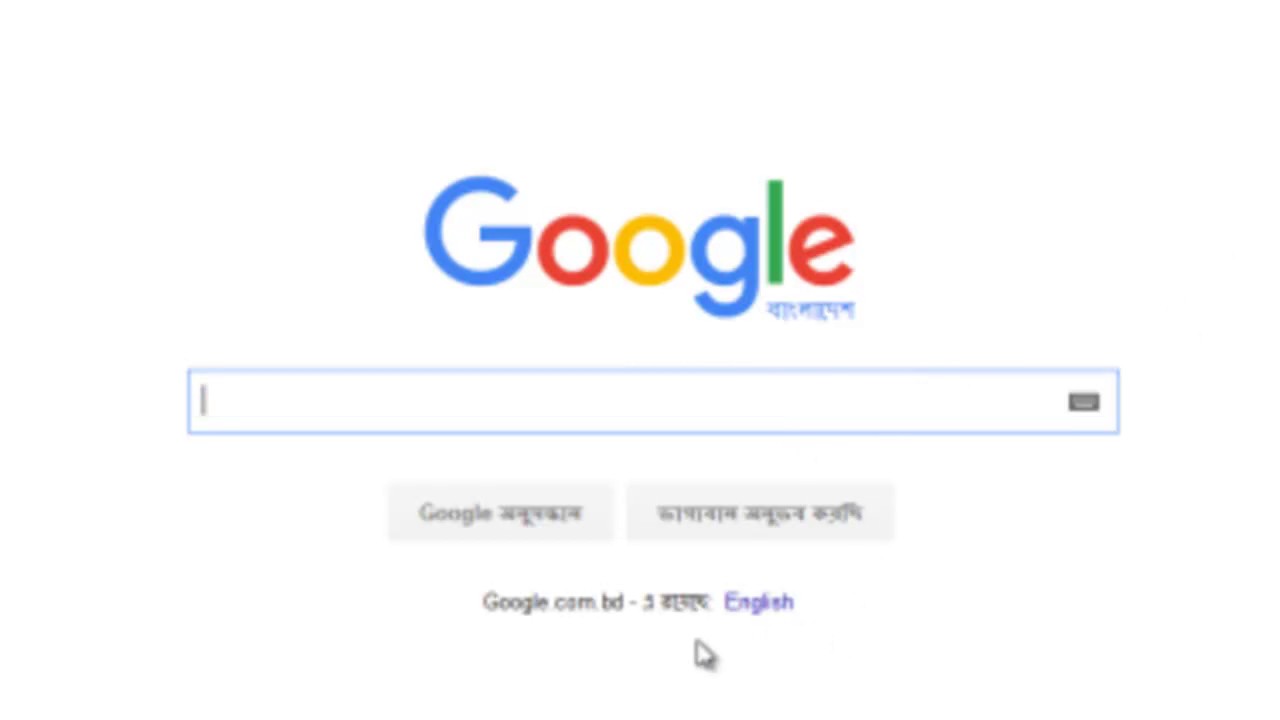The image depicts the Google search homepage tailored for an Arabic-speaking audience. Dominating the upper portion is Google's iconic large, blue "G" logo, followed by the letters "L-O-G-L-E" in the same distinct typeface. Below the logo, Arabic text is prominently displayed, signaling the primary language setting of this page. At the center of the page, there is a classic Google search input bar, flanked by light gray suggestion bars that hint at possible search terms. The bottom left of the page shows "Google.com" with an option to switch to English. The background is a clean, minimalistic white, making the input field and text stand out. This webpage showcases Google's familiar layout, both aesthetically pleasing and user-friendly, designed specifically for Arabic users as indicated by the "Google.com.bd" URL.